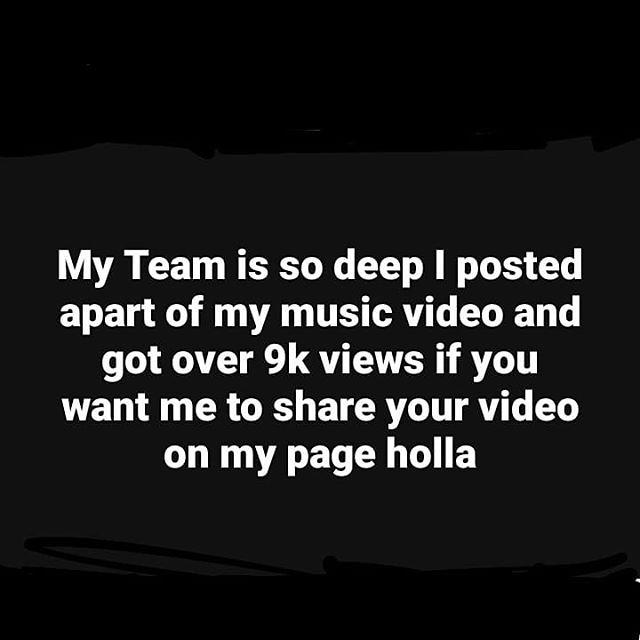The image features a message on a dark, artsy background. The top and bottom sections of the backdrop are black with jagged, hand-drawn edges, while the middle section is a lighter gray. The text, centered in the image, is in bold white font and reads: "My team is so deep I posted a part of my music video and got over 9k views. If you want me to share your video on my page, holla." The phrase "a part" is written as one word. The text spans five lines and is in regular, unembellished font. There are no punctuation marks at all. The bottom right corner shows a small white dot, possibly a remnant of whatever was originally covered by the black streaks.